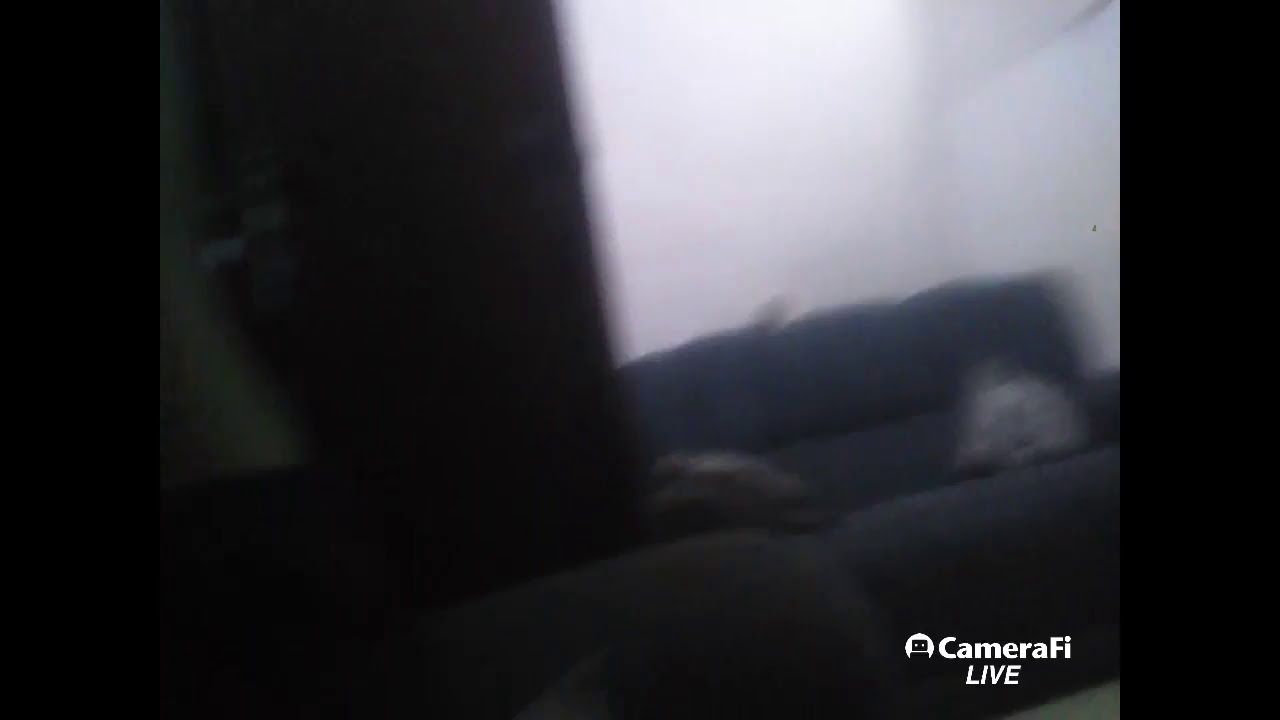The image is a blurry digital photograph, seemingly captured from a webcam or webcam feed, possibly using CameraFi Live, as indicated by the text in the bottom right corner. The scene is set in a dimly lit living room with a darker-colored couch, which appears blue, positioned in a corner against light-colored walls, likely white. The couch has a couple of pillows on it, one of which might be mistaken for a small cat. There are also two bags on the couch, a white one and a black and white one. On the right side of the couch, there appears to be a window. The left side of the image is obscured by a giant black blotch, and there might be a person's leg or arm visible, suggesting someone might be sitting nearby.